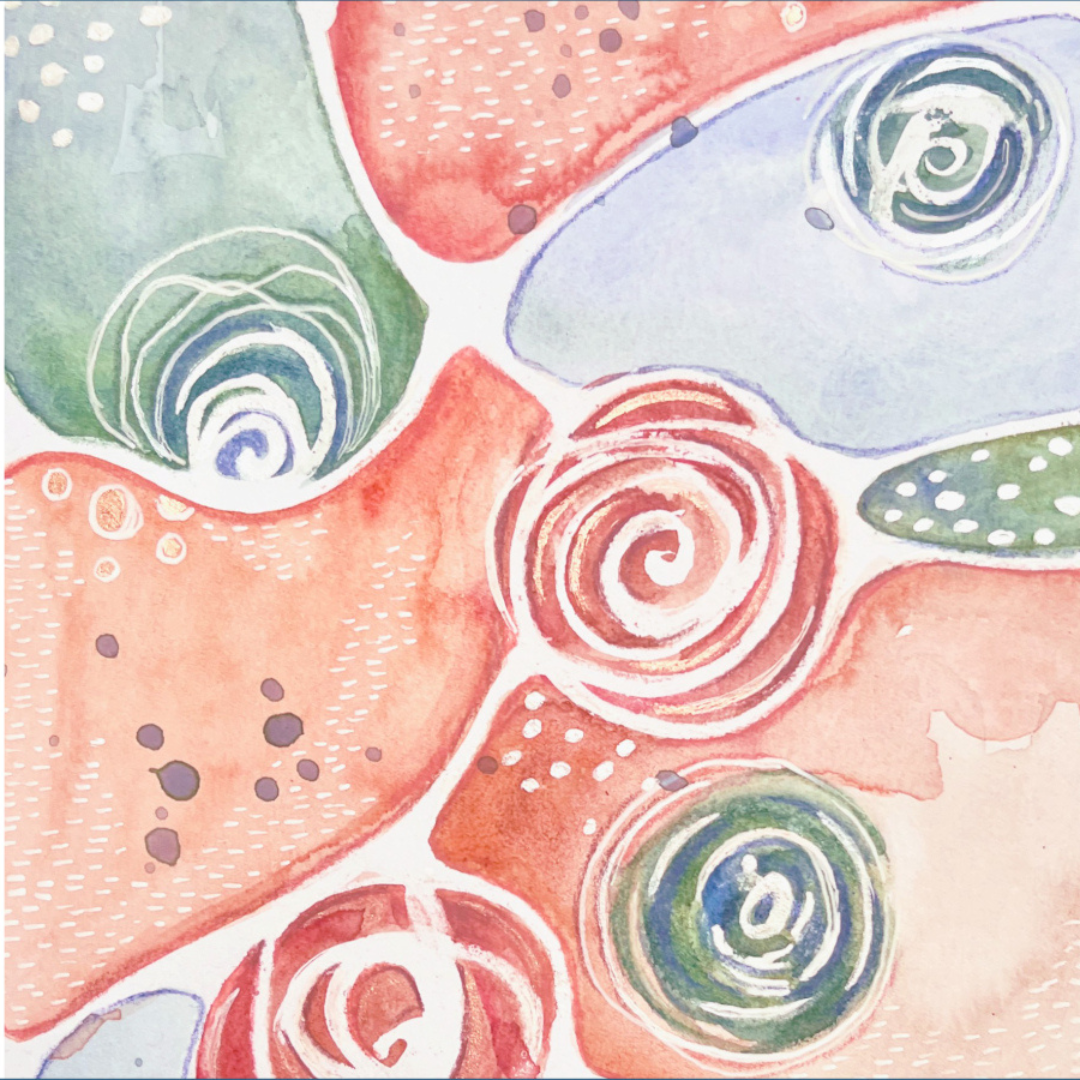This is an abstract piece of art featuring a vertically rectangular composition with no specific borders, set against a white background. The painting includes a dynamic mix of various colors like red, green, blue, and different shades of pink. At the center, there is a prominent swirl with lighter and darker pinks that resembles a rose. Surrounding this, there are multiple splotches of colors, each containing smaller swirl shapes in green and blue. These swirls of colors create floral-like patterns, interspersed with splashes and swatches that give the impression of paint being spilled. Despite its abstract nature, the piece has an intricate design, with each colorful swirl and shape separated by the white background.